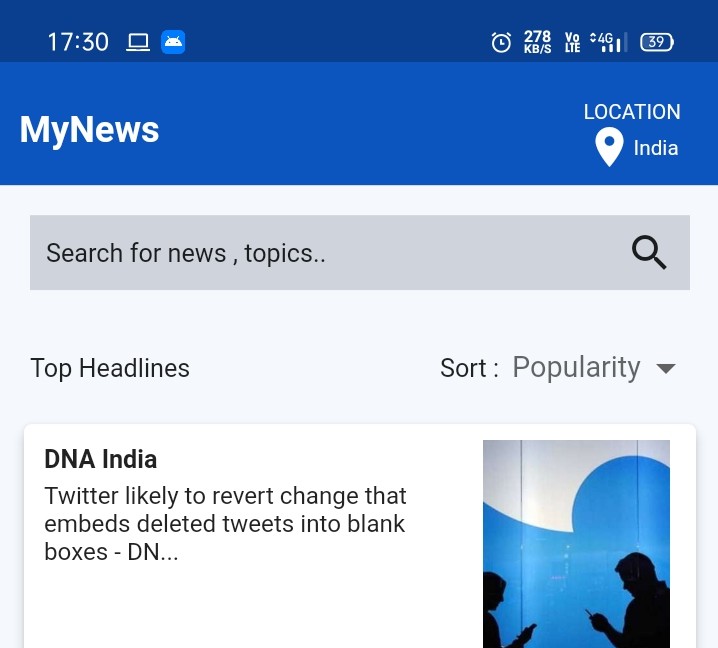The image is a squared screenshot from a phone, showcasing the top half of the screen. The top section of the image is dominated by a blue background. On the top left, in white letters, the time is displayed as 17:30. To the right of the time, there is a series of icons: a laptop, an Android logo, a large blue space, an alarm clock icon, and the download speed indicated as 278 KB/s. Further to the right, "VOLET" is displayed next to the 4G icon, showing three out of four bars of signal strength. At the far right, the battery icon reads 39%.

Below the time, on a lighter blue background, the heading "My News" is visible. Directly below the battery icon, "Location" is indicated. Next to it, a matte-tip white pen icon is labeled "India."

Below this lighter blue section, on a white background, a search bar prompts "Search for New Topics" with a magnifying glass icon to its right. Beneath this search bar, underlined by a white background as well, the section is titled "Top Headlines" with a sorting option labeled "Popularity" accompanied by a downward arrow.

The news headline from DNA India reads, "Twitter likely to refer to change that embeds tweets into blank boxes," flanked on the right by a square image. The image depicts a blue and white wall and the silhouettes of two people on their phones facing each other.